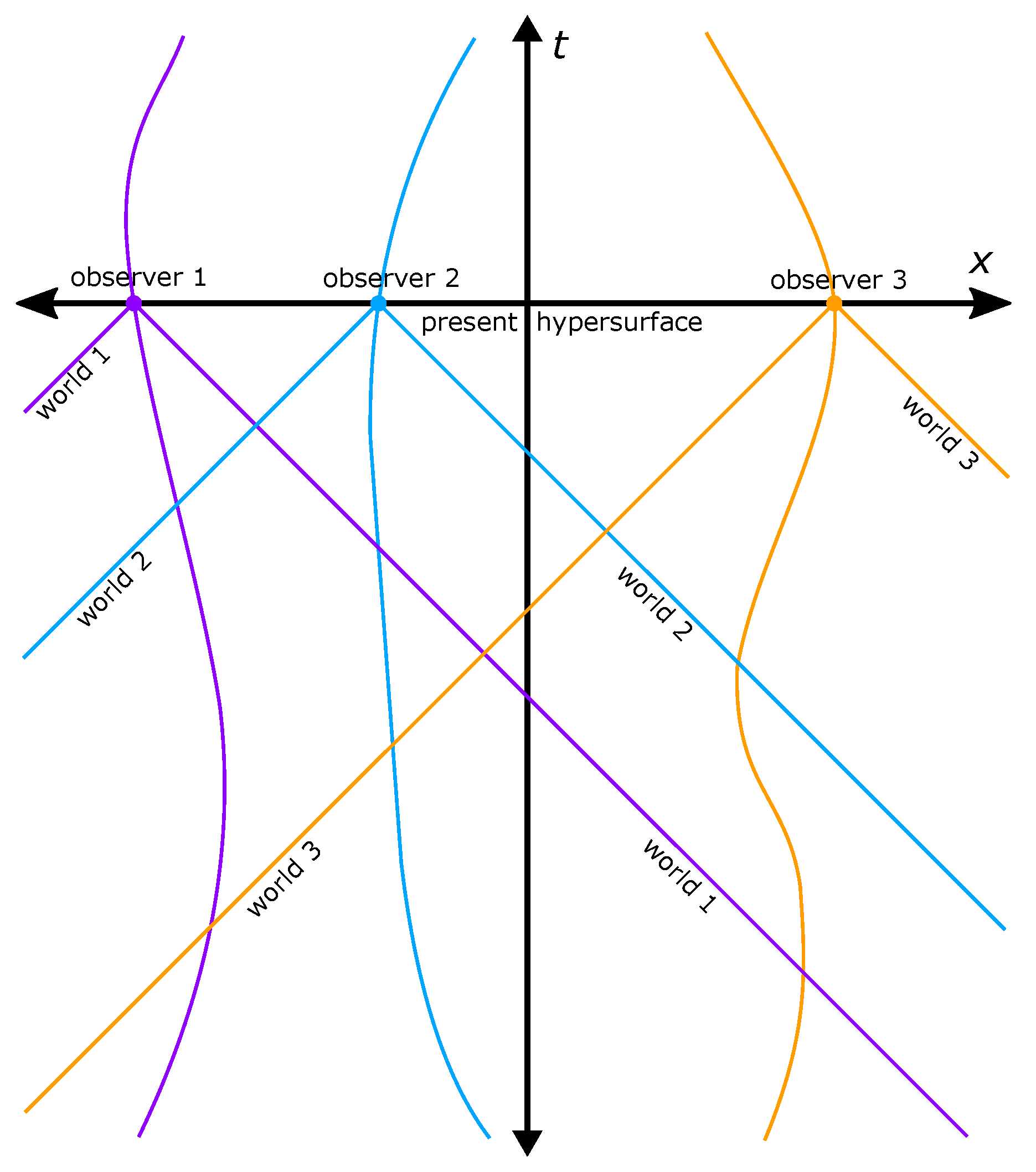This is an illustration with an X-axis and a Y-axis, intended to convey an informational or instructional concept about three observers. The X-axis features "Observer 1," "Observer 2," and "Observer 3" positioned from left to right. The Y-axis represents time, labeled as "T," and includes the term "Present Hypersurface." Each observer has three lines extending from their position: two straight lines and one wavy line. Observer 1's lines are associated with "World 1" in purple, Observer 2's lines with "World 2" in aqua blue, and Observer 3's lines with "World 3" in orange. These lines extend across both the X and Y axes, illustrating the different perspectives and times that each observer experiences, emphasizing the concept that our observations and interpretations vary based on our distinct viewpoints. The graphic predominantly uses a black and white color scheme, with the exception of the colored lines representing different worlds.